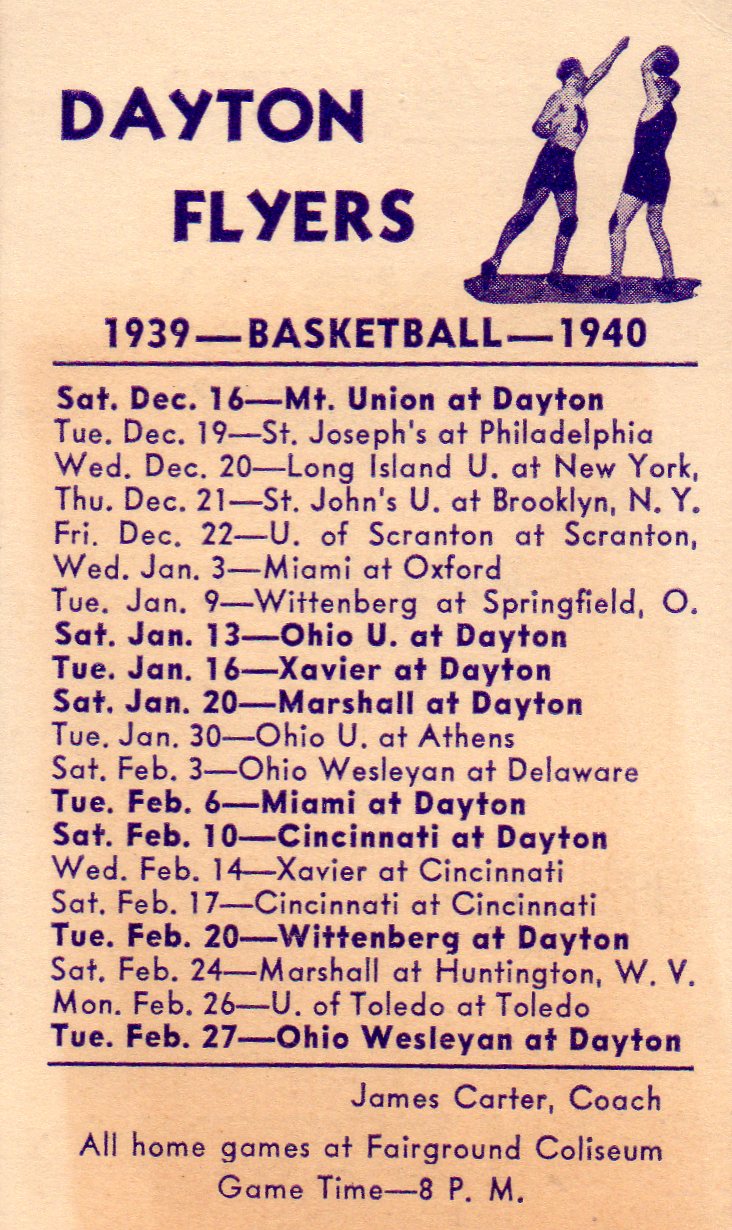This is a detailed poster of the 1939-1940 basketball schedule for the Dayton Flyers. The poster features dark print on a pink background and has a distinct vintage feel, resembling aged, beige paper that once might have been white. At the top, "Dayton Flyers" is prominently displayed in bold, dark blue letters, accompanied by an illustration of two basketball players on the right side. The player on the right, wearing a black jersey and shorts, is holding a basketball above his head, while the player on the left, clad in a white jersey and black shorts, attempts to block with an extended left hand.

Below the illustration, the text "1939/Basketball/1940" is underlined, followed by a detailed game schedule. The schedule starts on Saturday, December 16th, 1939, with Mount Union at Dayton and concludes on Tuesday, February 27th, 1940, with Ohio Wesleyan at Dayton. In total, the schedule lists approximately 20 games, including notable matchups like St. Joseph's at Philadelphia on December 19th, Long Island U at New York on December 20th, and Ohio Wesleyan at Dayton on February 27th.

At the bottom of the poster, it's noted that James Carter is the coach of the team. Additionally, it specifies that all home games will be held at the Fairground Coliseum, with game time set for 8 p.m.